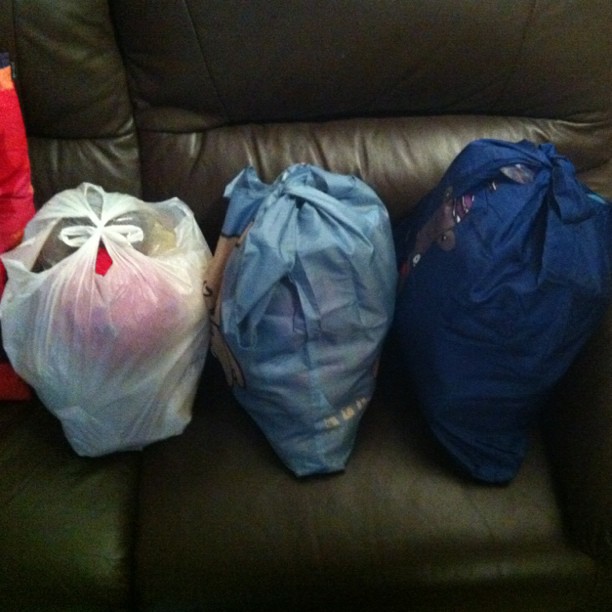In this square, slightly grainy, low-resolution color photograph, a dark brown and dark green faux leather couch is depicted with slight textural ruching on the backrest. The seating area is occupied by various bags that obscure the seating surface. 

On the far left edge of the frame is a sliver of a tall red bag or piece of material, potentially canvas. Next to it sits a well-filled white plastic grocery bag, tied at the handles, through which hints of red and other miscellaneous items can just be seen. 

Centrally positioned is a light blue translucent fabric tote bag with a beige design and some white lettering, also tied at the top, revealing indistinct dark shapes and some red contents within. 

To the right is a dark blue opaque tote bag featuring a character, possibly a brown or gray monkey, also tied at the top and appearing full.

This spread of bags atop the couch suggests a scene of organized clutter, perhaps indicating donation or transport preparations.